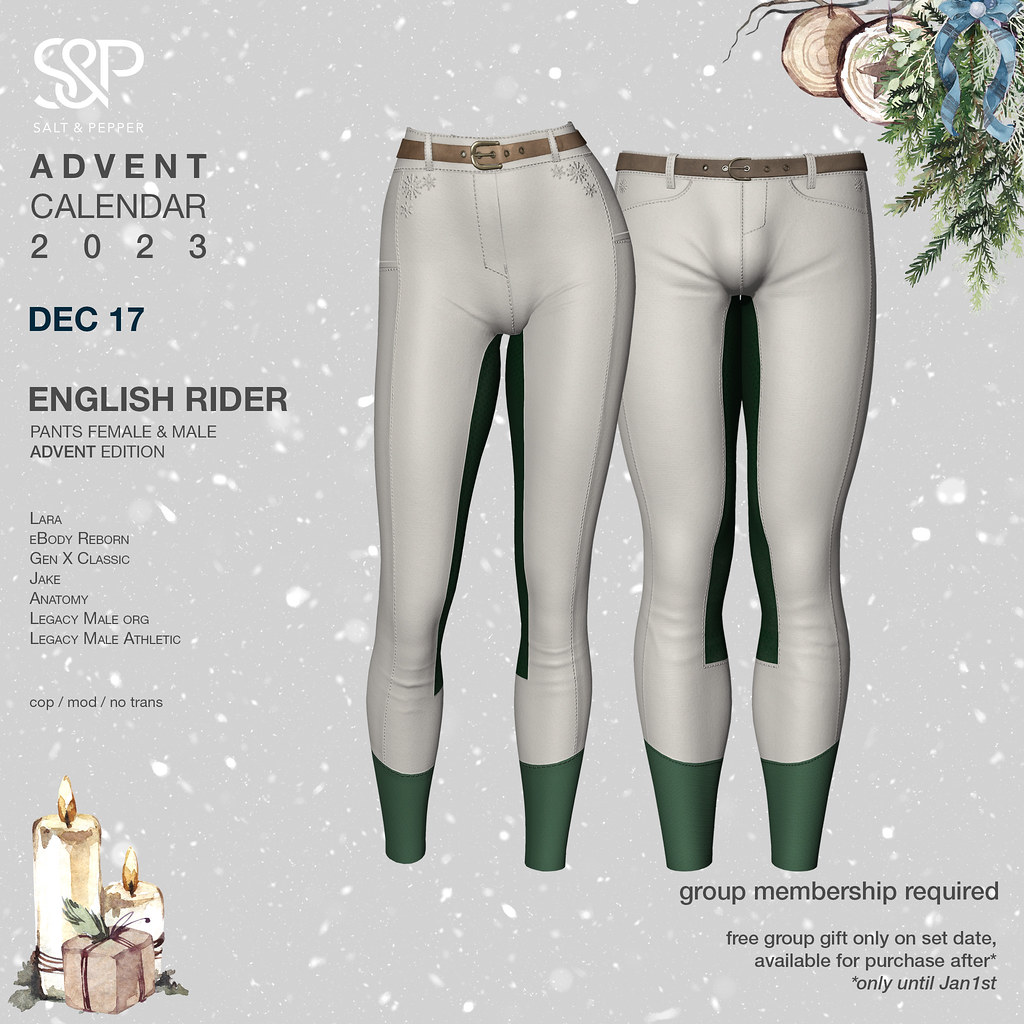The advertisement features an image showcasing a pair of male and female gray riding pants, identified as the "English Rider Pants Advent Edition." The pants come with a brown belt and feature a distinctive black stripe that runs from the crotch down past the knees, paired with matching gray socks. The background is a light blue color adorned with white dots resembling falling snowflakes, giving a festive winter ambiance. The top left and right corners prominently display “S&P Salt and Pepper” in a logo format. The top right also includes Christmas ornaments and mistletoe decorated with a blue bow. 

In the upper left corner, the text reads: "Advent Calendar 2023 December 17th English Rider Pants Female and Male Advent Edition." Associated product brands, such as Lara, eBody Reborn, Gen X Classic, Jake, Anatomy, Legacy Male Org, and Legacy Male Athletic, are listed below. The bottom left corner contains illustrations of candles and a Christmas present. The bottom right corner specifies, "Group membership required, free group gift only on set date available for purchase after only until January 1st."